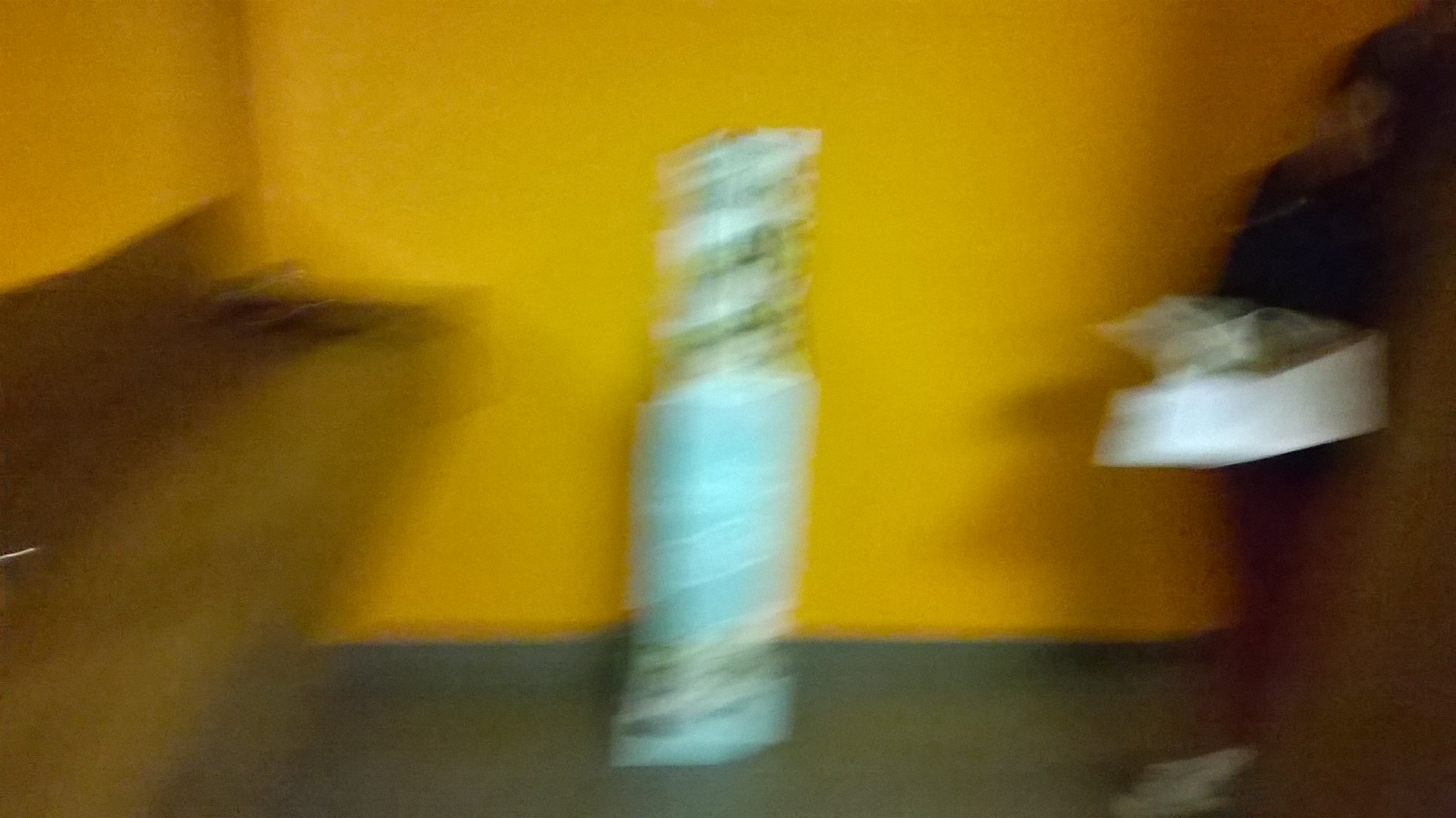This extremely blurry image depicts the corner of a room with dark golden marigold-colored walls and distinct black molding at the bottom. The floor is either dark gray or beige. On the far right side, there is a person standing, wearing a dark top and possibly with dark hair, though their features are indistinguishable. They are holding a large white object, possibly a plastic bin or tray, with pieces of paper on top. In the center of the image, there appears to be a large, light blue, cylindrical object with a spiral at the top, which some have described as a rectangular object with an indistinguishable picture or poster on it. On the left side of the room, there is a wooden shelf or counter mounted on the wall, featuring a dark object towards its end.